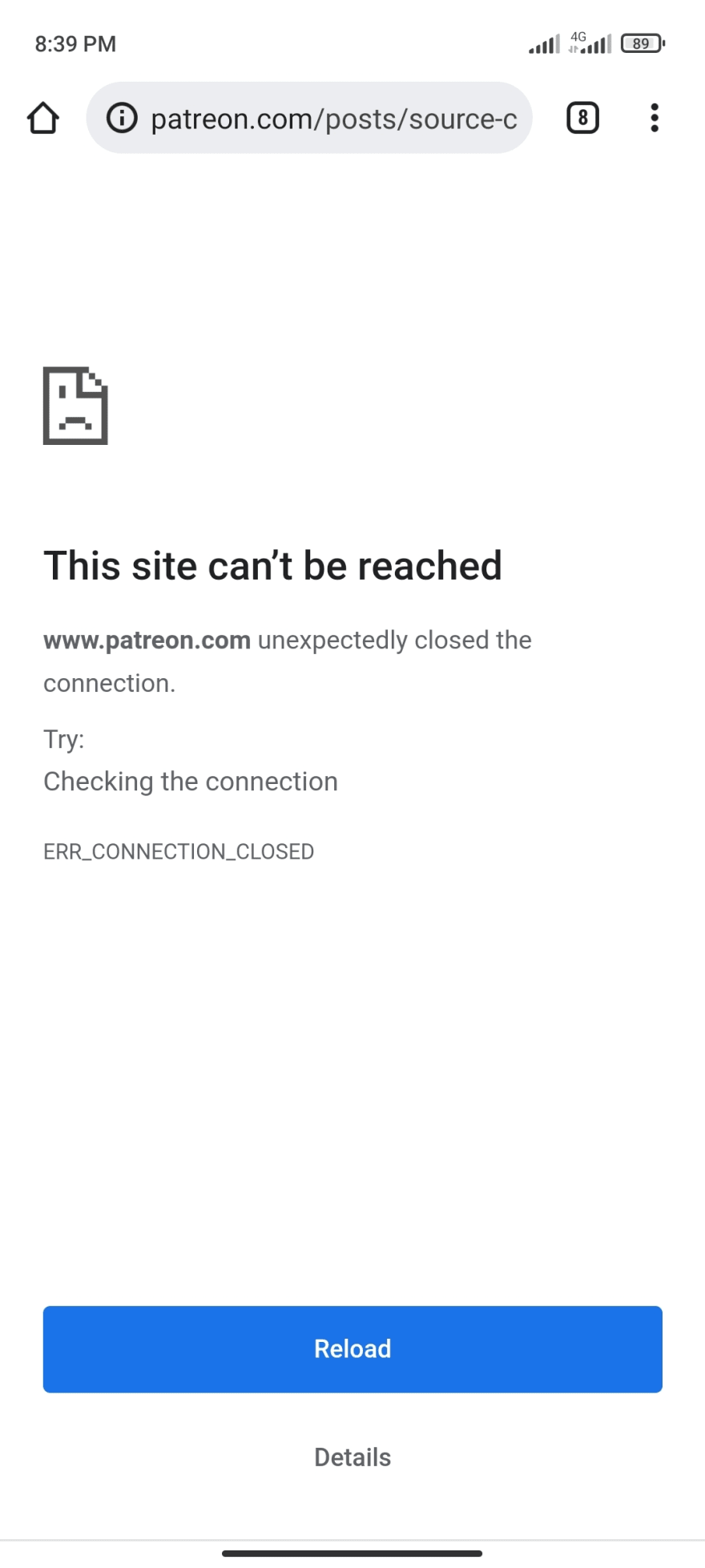A smartphone screen showing the time as 8:39 PM with the battery at 89%. At the top of the screen, a search bar displays an incomplete URL: "patreon.com/post/source-C...". Below this, an error message is presented with a frowning page emoji and the text, "This site can't be reached. www.patreon.com unexpectedly closed the connection." It advises, "Try checking the connection," and details an error code: "ERR_CONNECTION_CLOSED." Two buttons, labeled "Reload" and "Details," are shown underneath the error message, indicating an attempt to access a Patreon page that was unsuccessful.